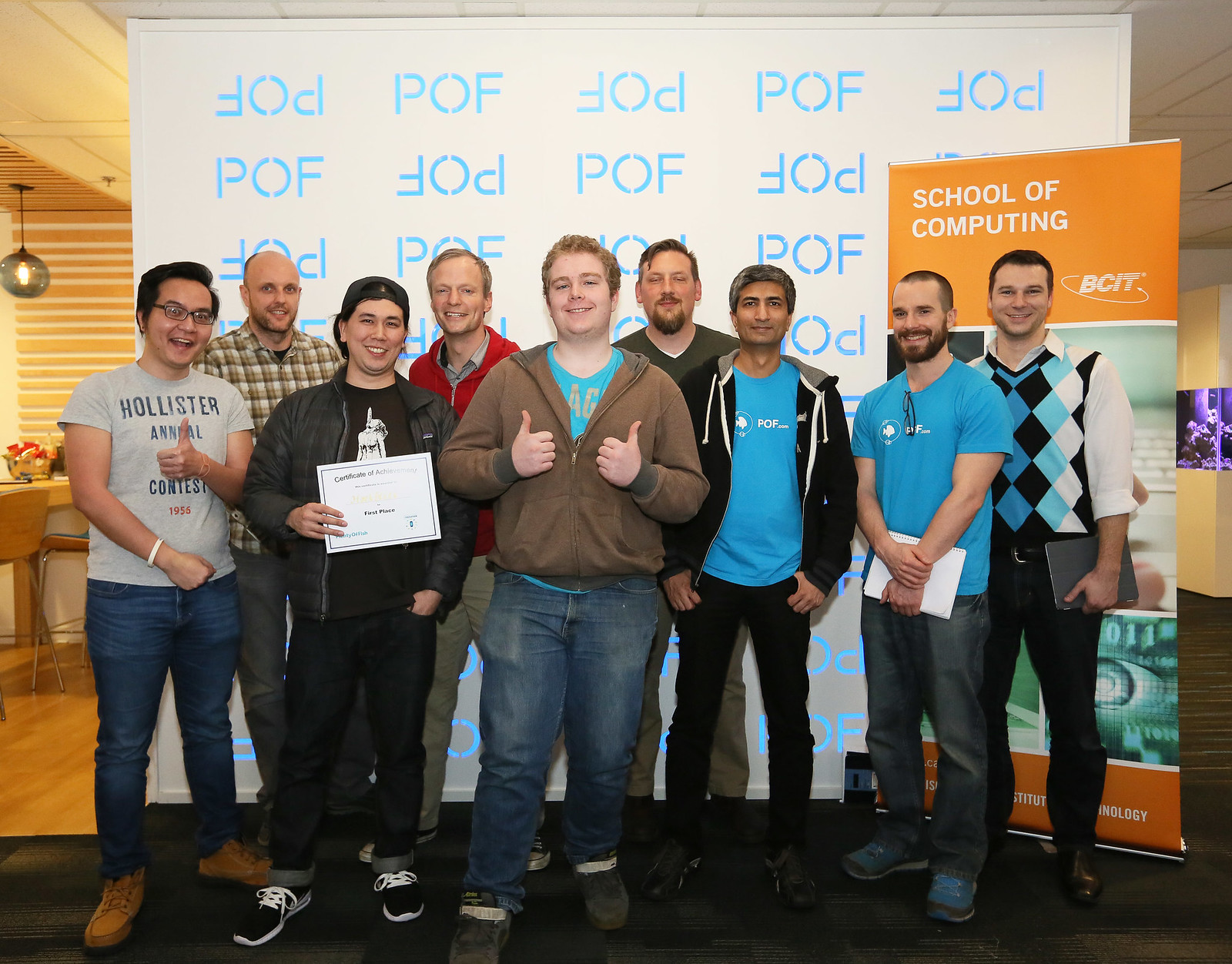This photograph captures a celebratory moment featuring a group of approximately nine adults and a couple of younger individuals, standing together and posing in front of a whiteboard repetitively displaying "POF" in blue, uppercase letters with a distinctive font. Behind them, an orange and white poster prominently reads "School of Computing" and includes the acronym BCIT, encircled by what appears to be an orbiting design. The group appears to be in a room with hardwood floors and yellow-painted walls, adjacent to a kitchen area equipped with a table, a bouquet of flowers, a hanging lamp, and a wooden chair with a green seat cushion. One individual in the group is seen holding a certificate, suggesting a special occasion, likely a graduation, with friends smiling and giving thumbs up in congratulations. Most group members are casually dressed in jeans, hoodies, jackets, or blue POF shirts, while one person on the far right wears a cardigan and a white long-sleeve shirt. The overall atmosphere of the photo is one of camaraderie and achievement.